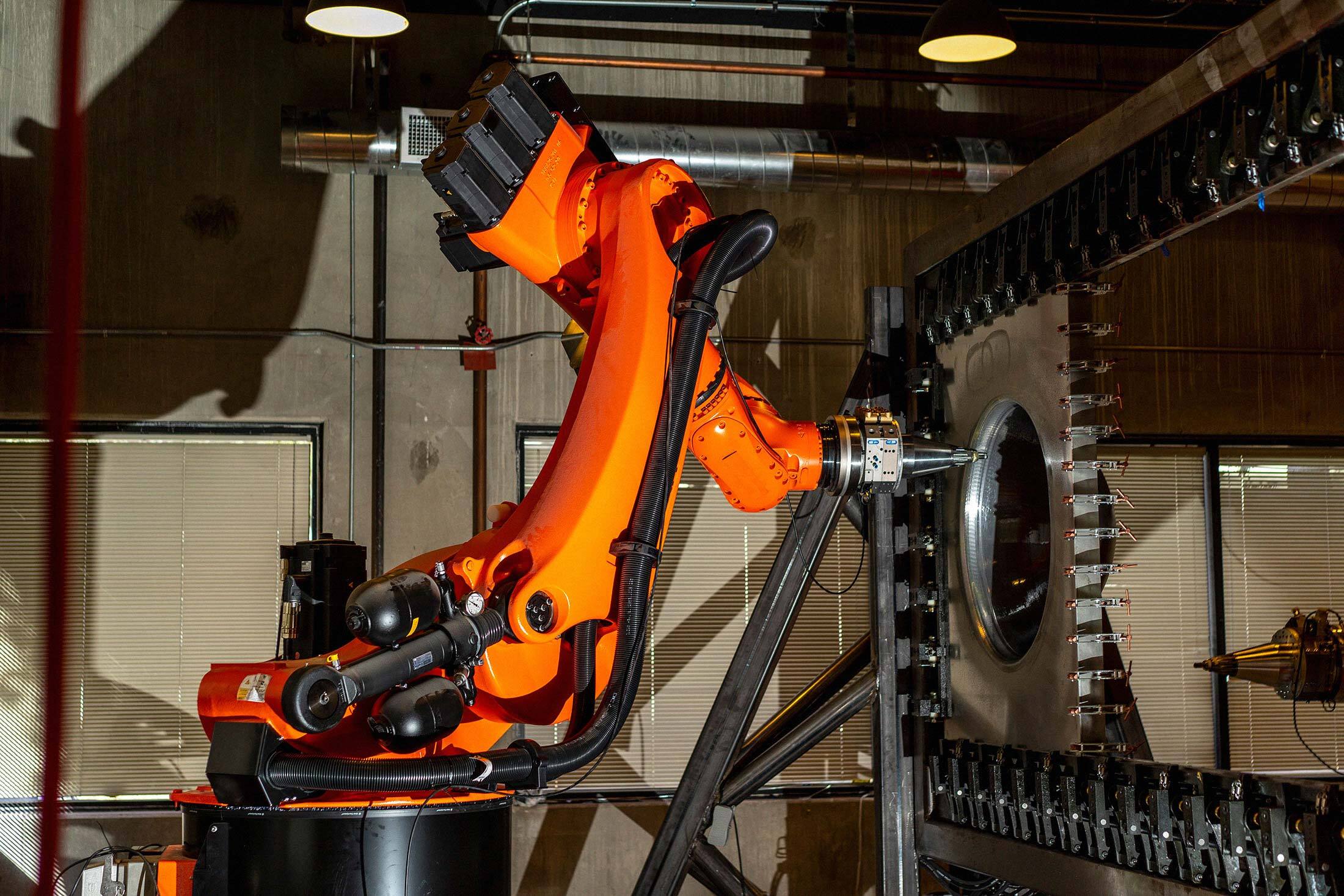The image showcases a high-tech, automatic hydraulic mechanical device primarily colored in orange. It has a distinctive, unusual shape—long, skinny, and resembling the letter "T." The device appears to be a sophisticated piece of machinery designed for precise, possibly delicate, metal work or drilling. The black hydraulic hoses and pumps are integral to its operation, suggesting its capability in performing repairs or industrial tasks. The machine is anchored at its base to a black drum and extends upward in an arc to the right. At the top, it features additional connecting mechanisms before descending again, ending in a pointed tip directed towards a large hole surrounded by metal, likely where its operative function takes place.

The setting is an industrial environment with gray walls featuring brown stripes and a background with lightly tanned window blinds. At the top of the image, there is a white light on the left and a yellow light on the right, highlighting the modern, high-end nature of the machinery. The image suggests the device's sophistication and advanced technology, capturing its detailed components, including lines and cables, in a very high-quality shot.